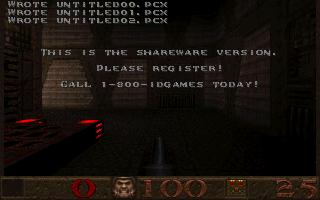This screenshot from a video game prominently features an almost entirely black background with faint light reflections off objects resembling walls. In the upper left corner, white text in all caps reads "WROTE UNTITLED 00.PCX". Directly below, the same font continues with "WROTE UNTITLED 01.PCX" and "WROTE UNTITLED 02.PCX". Centered across the image, white text announces, "THIS IS THE SHAREWARE VERSION, PLEASE REGISTER. CALL 1-800-ID-GAMES TODAY." At the very bottom of the screen, there is a status bar, likely indicating player health and stats. The bar displays a red "0", followed by an icon of a man's face, next to which is a "100" in a copper color. To the right of this is another indistinguishable icon, concluding with the number "25" also in the same copper color, located in the lower right corner.